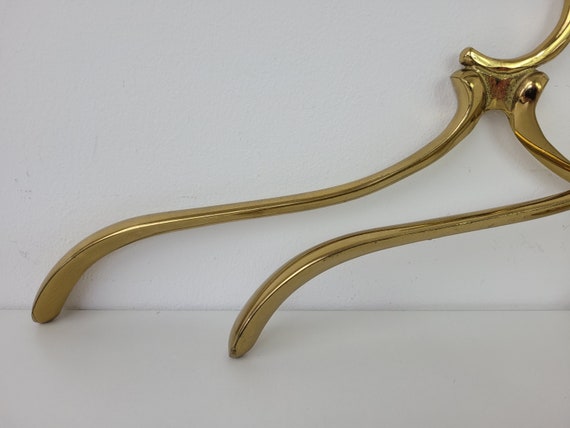The photograph features two smooth, golden brass coat hangers positioned on a white surface, against a white wall. The image captures only the left portion of each hanger, with the recognizable hook section visible on the right side but cut off from the frame. The hangers' flowing, almost wavy shapes create an abstract, swirling pattern that starts from the top right and extends down to the bottom left towards the center of the image. The glossy finish on the brass hangers reflects light, emphasizing their metallic and smooth texture. Despite their practical function, the arrangement gives off an impression of abstract art, leaning freely against the backdrop without any obvious support.